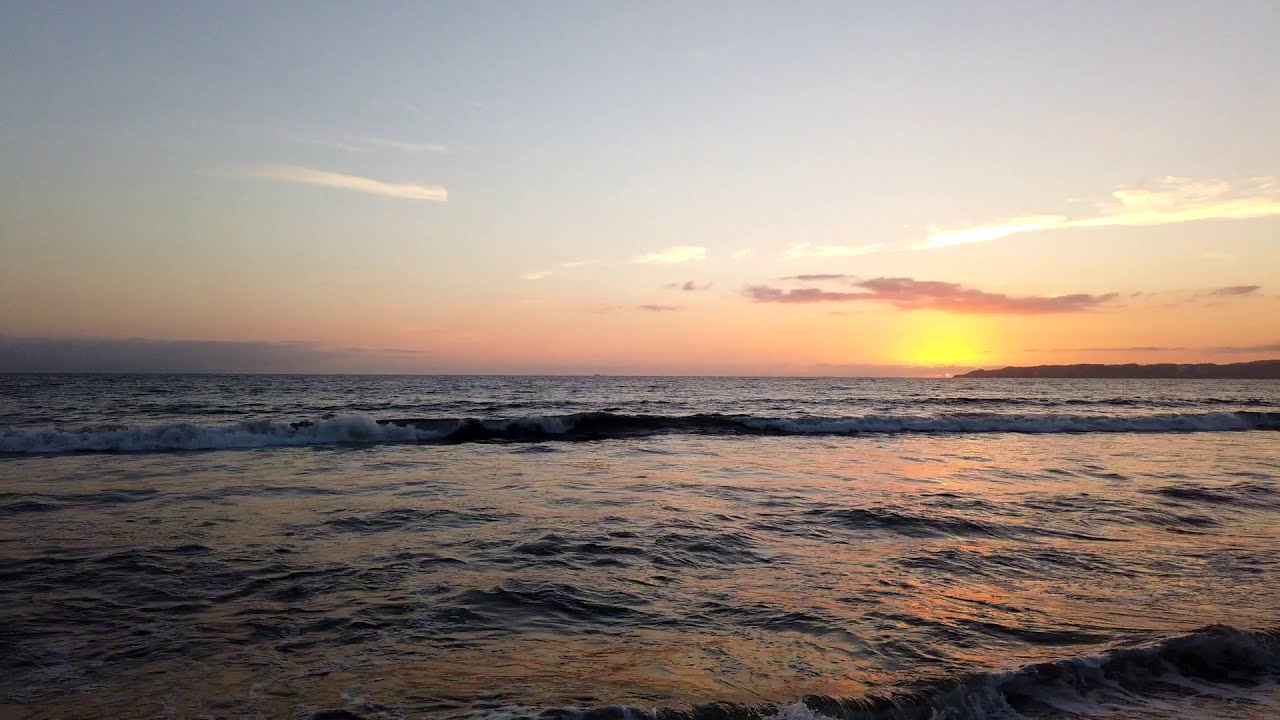This image captures a stunning beach scene at sunset, where the absence of sand draws focus to the tranquil ocean waves and the vibrant sky. The foreground is dominated by calm, rolling waves reflecting an array of warm sunset hues, including soft oranges, pinks, yellows, and deep blue tones from the water. The sky is a captivating gradient of yellows, pinks, oranges, and blues, with only a few delicate clouds, tinted in pinkish-blue, scattered above. On the horizon, the nearly set golden sun casts a reflective glow on the rippling water, enhancing the serene ambiance. The view is slightly angled, and off to the center-right, distant land formations, possibly rugged cliffs or mountains, just barely intrude into the scene, adding a picturesque detail to the expansive ocean and colorful sky.